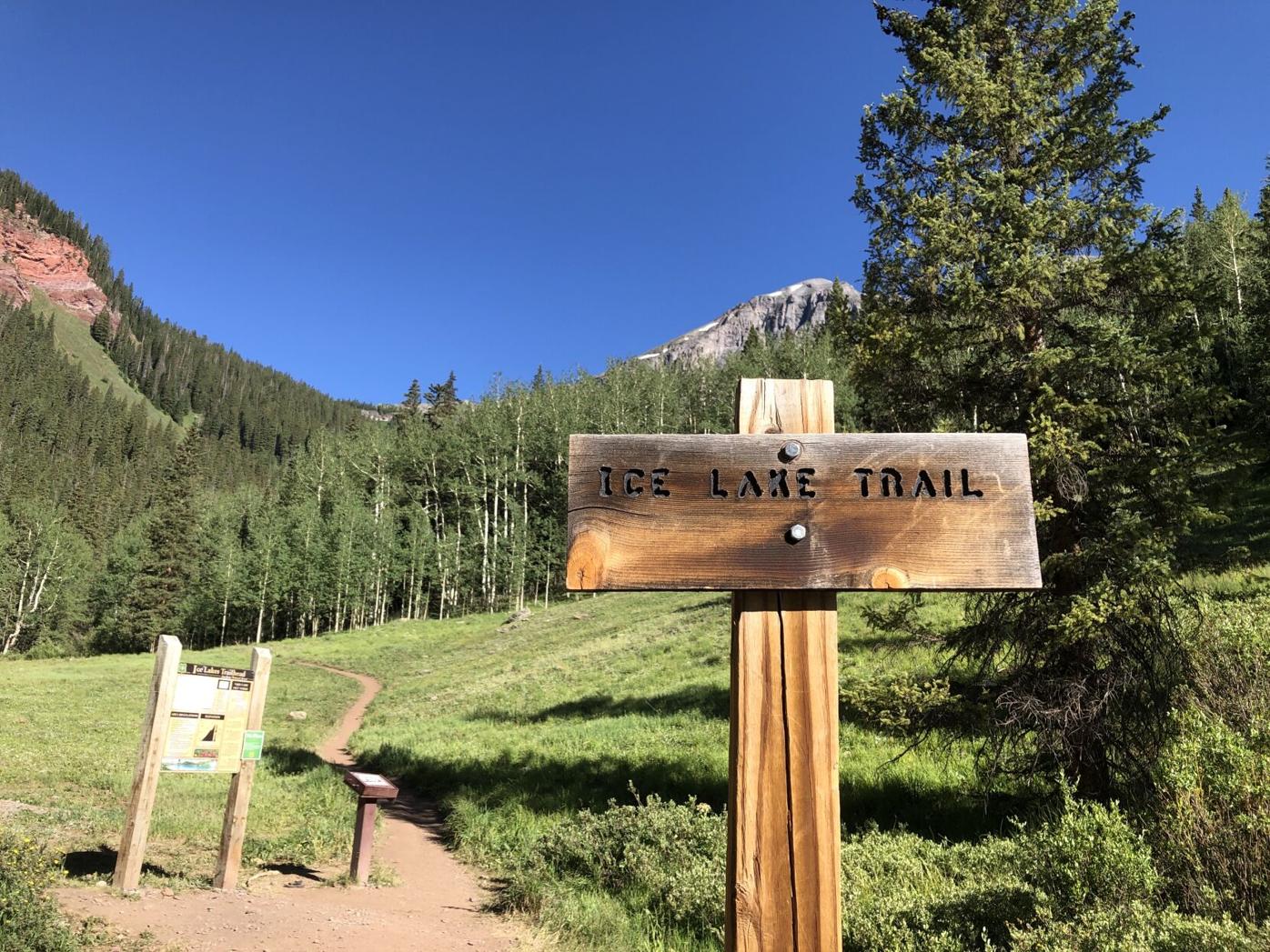This captivating outdoor photograph showcases a serene wilderness scene set deep within the woods. In the foreground, a sturdy wooden post stands tall, displaying a charmingly rustic sign with carved lettering filled in black paint that reads "Ice Lake Trail." The trailhead is indicated by a narrow dirt path that meanders off into the verdant forest, lined on either side by lush green grass. A tall green pine tree is perched above the right corner of the sign, while an abundance of slender tree trunks with bright green foliage frames the middle of the scene. In the background, majestic mountains capped with a hint of snow rise against the horizon, all beneath a flawlessly clear, bright blue sky. The vibrant colors — the greens of the trees and grass, the browns of the wooden sign and dirt trail, and the brilliant blue of the sky — come together to create a picturesque and inviting entry to the Ice Lake Trail.